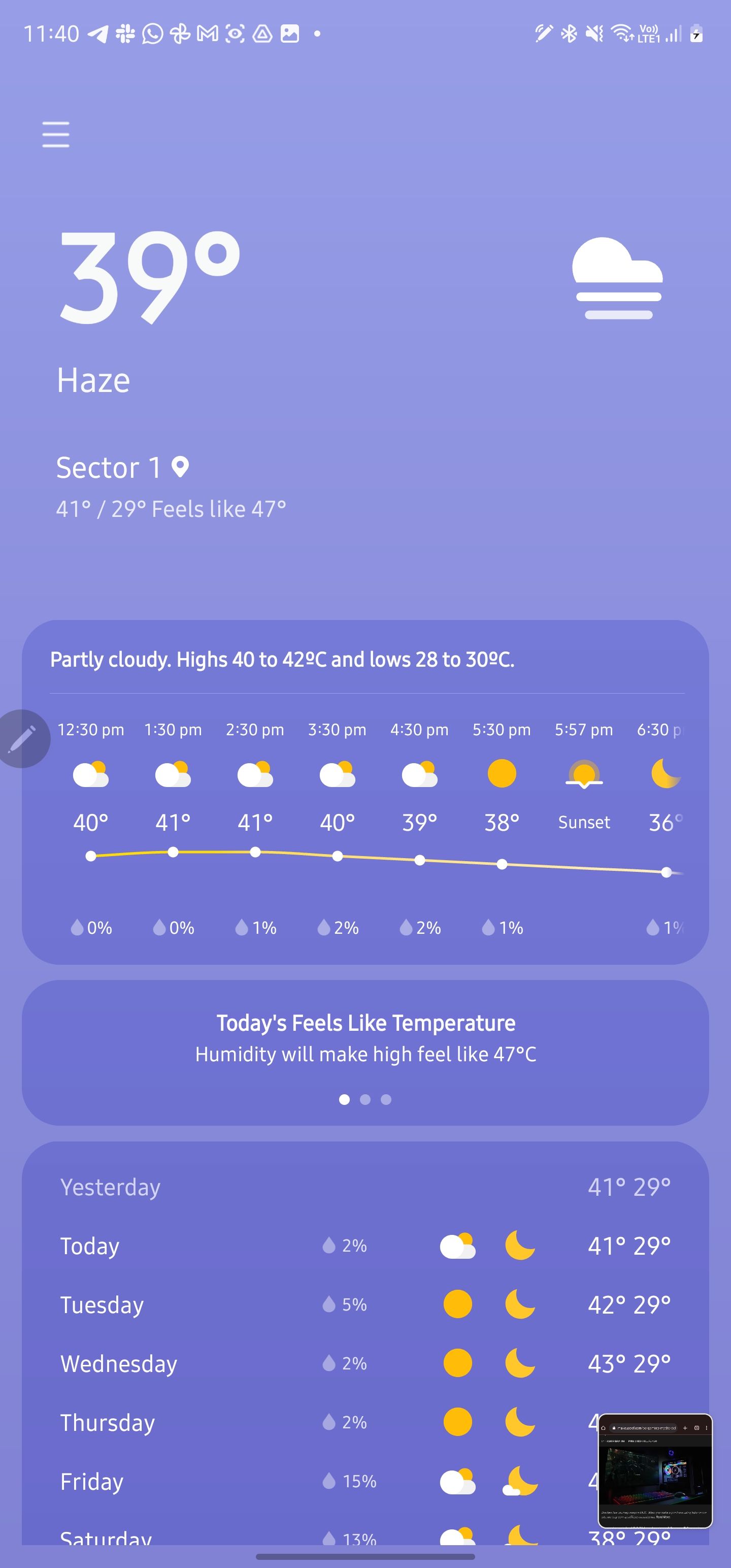The screenshot displays a smartphone with a lavender background. In the upper left corner, it shows the time as 11:40. The phone has several active icons, but the signal strength bars appear minimal, and the power level icon indicates roughly 50% remaining battery, though it is quite small. Additionally, the phone is on mute.

A hamburger menu is located on the left side, presumably for additional options. The screenshot centers on a weather application. It indicates a current temperature of 39 degrees, most likely in Fahrenheit. The weather icon depicts a mix of clouds and sun, with a note of hazy conditions. The high for the day is projected to be 41 degrees, with a low of 29 degrees. Although the current temperature feels like 47 degrees.

A temperature timeline forecasts a range from 40 degrees at 12:30 PM to 41 degrees later in the afternoon, eventually dropping to 36 degrees by 6:30 PM. The bottom of the screen provides historical data, showing yesterday's high and low were 41 and 29 degrees, respectively. The forecast extends through the upcoming days, from Tuesday to Saturday, detailing expected weather conditions.